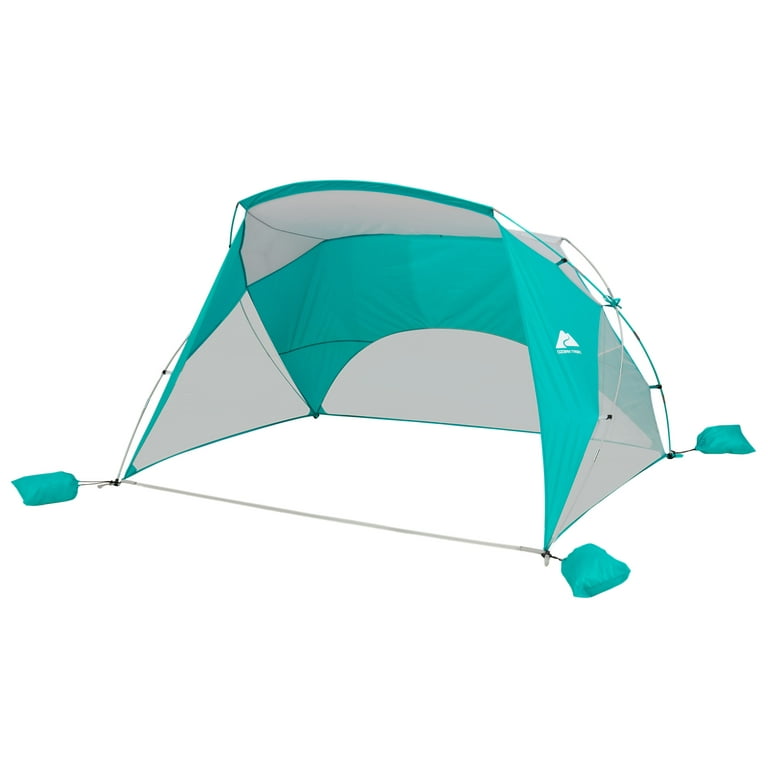The image showcases a beach canopy set up against a plain white background, highlighting its beach-themed colors of white and seafoam green. The canopy features a dome-like structure with an open front, providing a welcoming entry space. Each corner of the rectangular base is anchored by seafoam green sandbags, ensuring stability in breezy beach conditions. This practical design helps prevent the canopy from blowing away. The canopy includes a subtle white logo on one of the seafoam green panels, depicting a stylized mountain with a curving road, although the accompanying text is not legible. The entire setup is user-friendly, emphasizing ease of transport, assembly, and disassembly, making it an ideal choice for creating shaded refuge during a day at the beach.